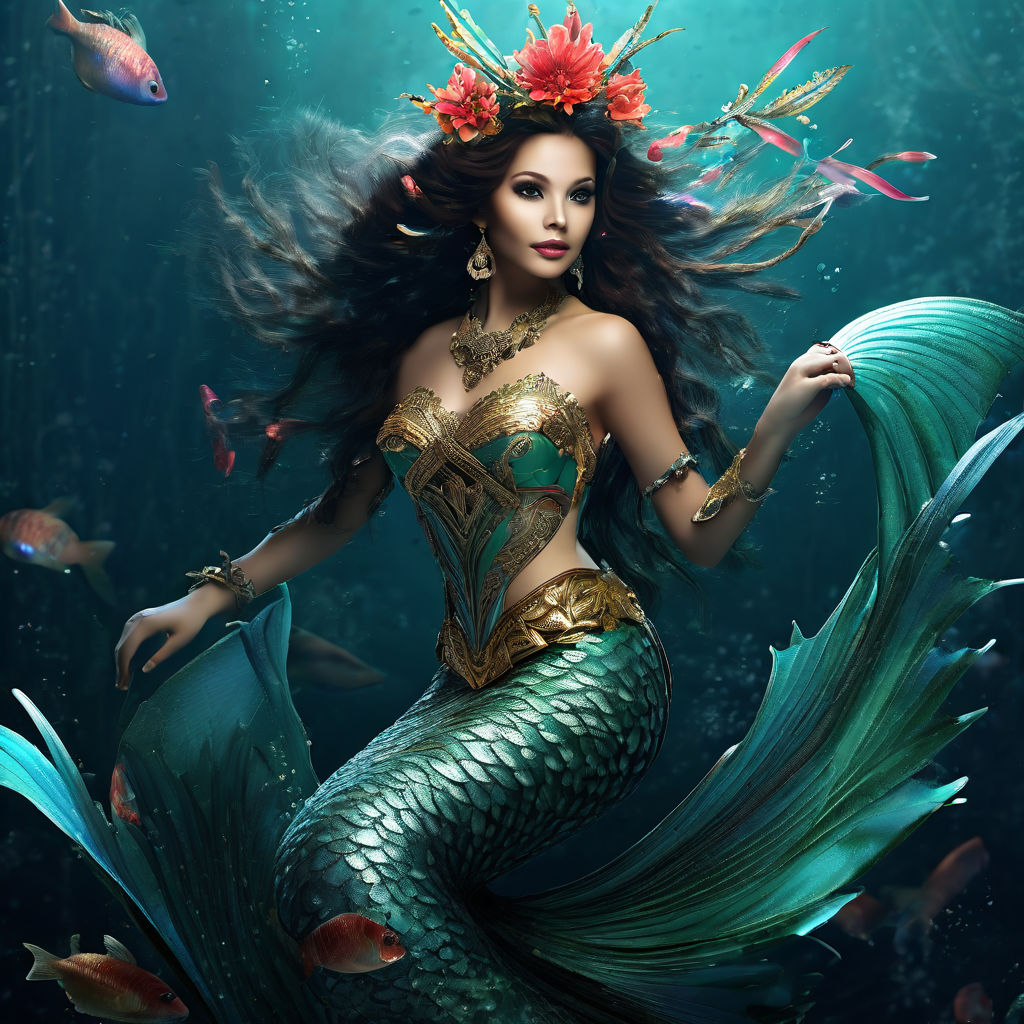This is a detailed and realistic digital illustration of a mermaid, set against a deep blue underwater background. The mermaid's upper body resembles that of an elegant woman, adorned with black, flowing hair decorated with a red flower crown. Her attire is intricate, featuring a green and gold breastplate, an elaborate bronze and gold necklace, a golden belt, and various bracelets and rings on her hands. Her lower body's fish tail is covered in shimmering silver scales. The mermaid is looking slightly to her right, exhibiting a futuristic and airbrushed appearance. Surrounding her in the water are swimming fish, adding to the animation-like quality of the image. The entire composition is presented in a square format, giving the artwork a balanced and symmetrical feel.